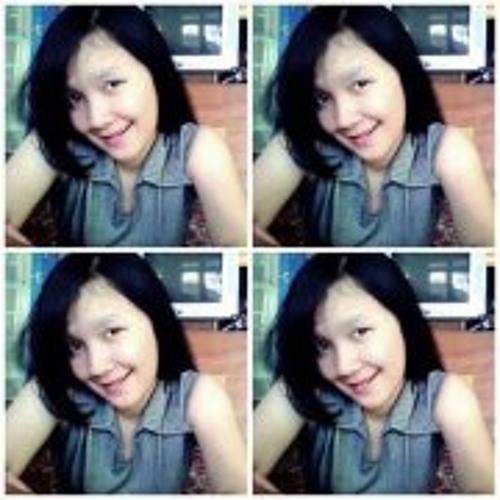This image is a series of four identical photos arranged in a windowpane style, separated by a narrow white border. The photos feature a dark-haired woman with shoulder-length hair, wearing a blue sleeveless shirt, and are captured from the chest up. In each photo, her head is slightly slanted to the side. The background includes a TV in the upper right corner and a wood-toned floor. The colors present in the image are brown, black, yellow, pink, and red. The entire set of photos seems to be personal snapshots taken by someone, exhibiting a cozy and casual atmosphere without any text.